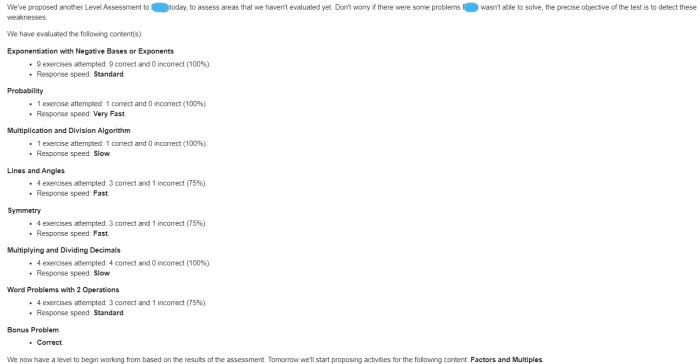The image contains a white background covered with black text, resembling a webpage displaying a message for an individual in a specific role. At the top, there's an introductory statement: "We proposed another level assist assessment to [BLANK] today by [BLANK]"—the names have been obscured using a blue editing tool. The text explains the purpose of the assessment is to evaluate previously unexplored areas.

The text reassures, "Don't worry if there are some problems," noting that "[BLANK] wasn't able to solve the precise objective of the test," which is to identify weaknesses. It then lists the areas evaluated in the assessment, each heading is bolded followed by bullet points:

1. **Exponentiation with Negative Bases or Exponents**
2. **Probability**
3. **Multiplication and Division Algorithm**
4. **Lines and Angles**
5. **Symmetry**
6. **Multiplying and Dividing Decimals**
7. **Word Problems with Two Operations**
8. **Bonus Problem**
   - Correct

At the bottom, the message concludes, "We now have a level to begin working from based on the results of the assessment. Tomorrow we'll start proposing activities for the following content: factors and multiples."